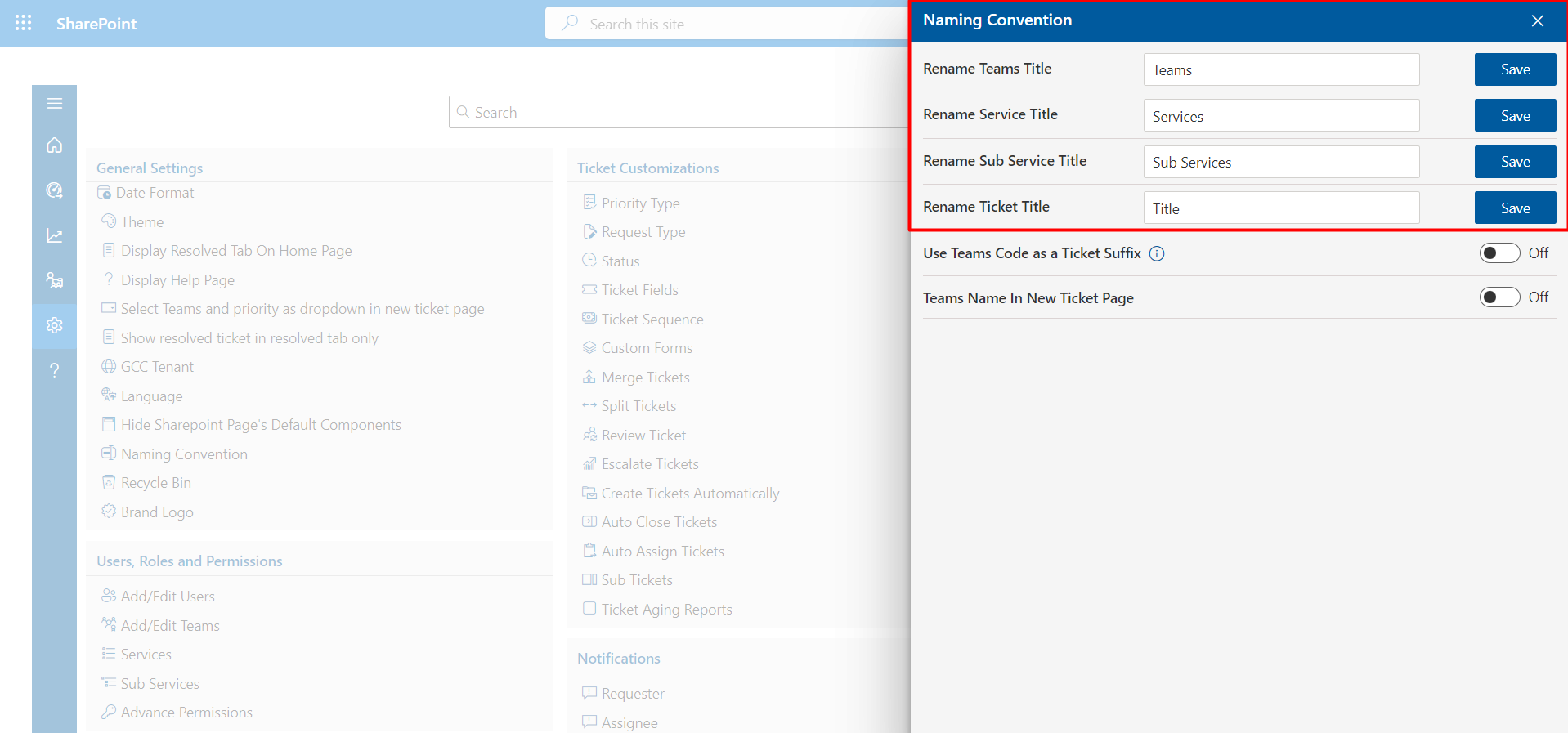This is a detailed screenshot of the SharePoint app interface. The left portion of the screen is grayed out, directing focus to an active modal window on the right side, which is outlined in red for emphasis. At the top of this Window's modal, the title "Naming Convention" is prominently displayed. Below this, four text fields are sequentially organized:

1. **Rename Teams Title**: The text field contains "Teams".
2. **Rename Service Title**: The text field reads "Services".
3. **Rename Sub-Service Title**: The text field shows "Sub-Services".
4. **Rename Ticket Title**: The text field displays "Title".

Next to each text field is a "Save" button, characterized by white text on a blue background. Below these, two additional settings are present:

- **Use Team Codes as a Ticket Suffix**: Accompanied by a toggle button, currently set to "Off".
- **Team's Name in New Ticket Page**: This also has an adjacent toggle button set to "Off".

This comprehensive layout facilitates customization of titles within the SharePoint application, streamlining user experience with clearly marked save options and toggle settings.